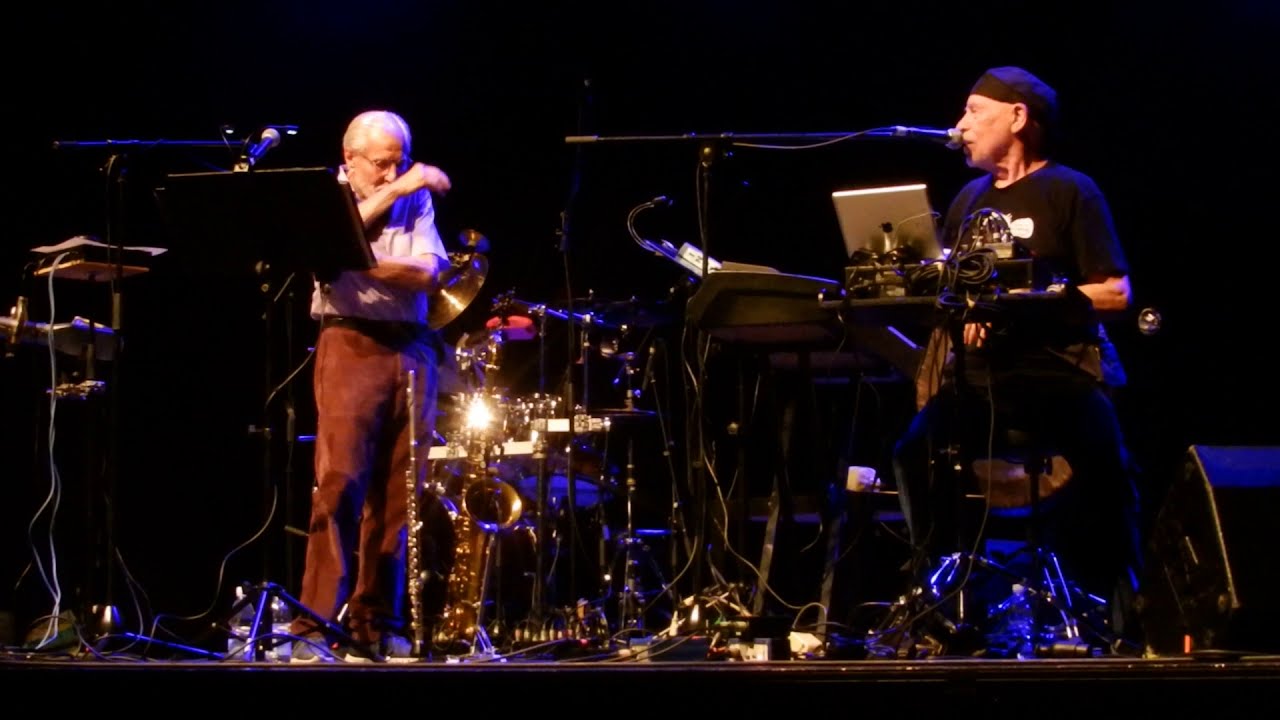The image captures a live music performance featuring two older men on stage against a dark background illuminated by a spotlight, which casts a blue hue reflecting off their instruments. On the left, a man with gray hair and eyeglasses clad in a white short-sleeve shirt and brown pants stands with his arms raised, gesturing animatedly. He is positioned in front of a black podium holding sheet music and a microphone. To his right, another man is seated, wearing a black t-shirt and a black hat, speaking into a microphone positioned close to his mouth. In front of him rests an Apple laptop and a keyboard. The stage setup includes various instruments such as a saxophone and a flute on stands, a drum set, and a keyboard, with the saxophone notably reflecting the stage lights.